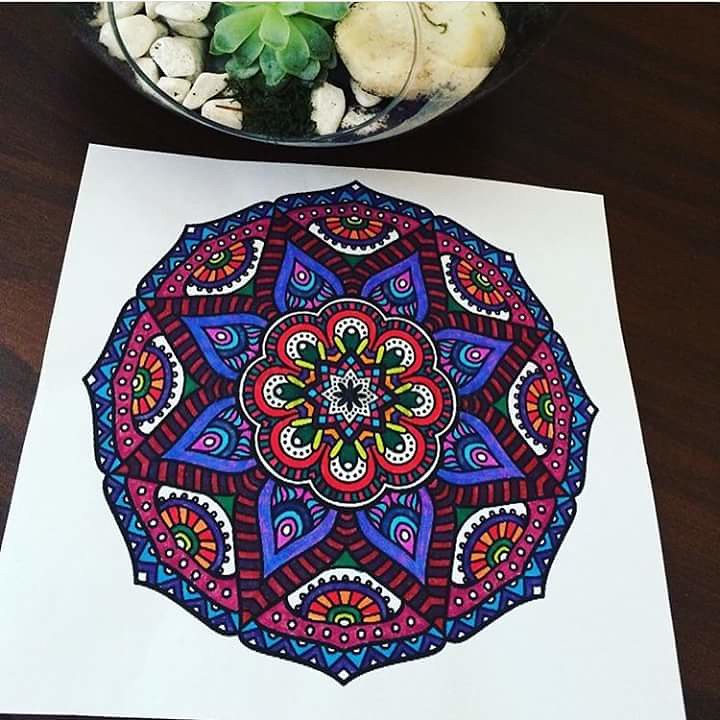The photograph captures an intricate, vibrant drawing on a white square piece of paper, placed on a dark brown wooden table. The artwork features a complex, symmetrical design reminiscent of Indian or Asian patterns, with a central floral motif radiating outward like a kaleidoscope. The dominant colors are red, blue, light blue, purple, yellow, and orange, creating a hypnotic, fractal-like composition with floral and petal shapes. Surrounding the central flower-like shape, the design incorporates inversed hearts, triangles, and semi-circular patterns, all meticulously detailed in an elegant arrangement. 

In the top section of the photograph, a glass container is visible, housing a small, green succulent set among white rocks, a significant large white stone, and brown dirt, adding a natural element to the scene. The combination of the detailed artwork and the verdant mini terrarium creates a visually captivating and harmonious composition.